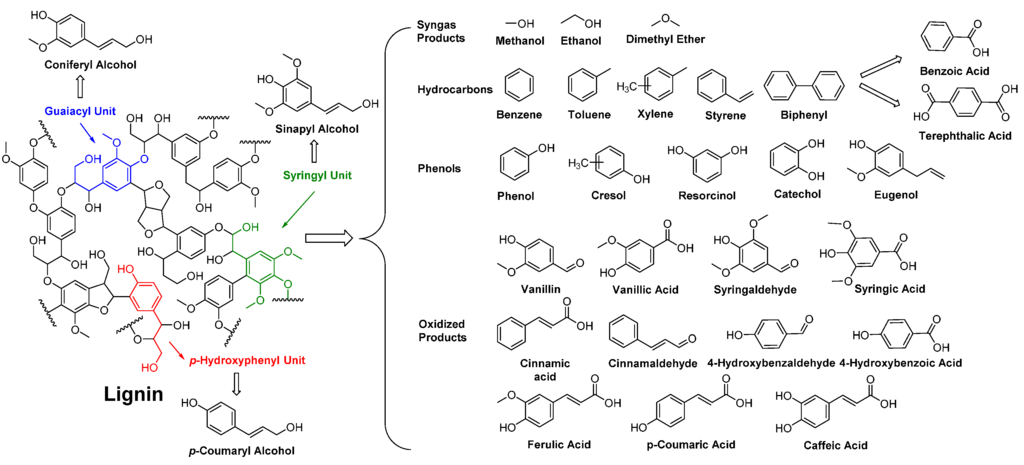The image is a detailed landscape-oriented diagram showcasing the breakdown of the complex molecule lignin and its subsequent chemical reactions. At the top left, the word "Lignin" is prominently displayed in bold black letters, signifying the starting material. Surrounding this are a network of interconnected molecular compounds, illustrated in various shapes and colors, each with names and arrows indicating the progression of reactions. Key compounds include:

- P-hydroxaphenyl unit (red) converting to P-coumaryl alcohol.
- Syringyl unit (green) converting to synapyl alcohol.
- Glycol unit (blue) converting to coniferal alcohol.

As these compounds react, they form various intermediates before breaking down into smaller products such as methanol, ethanol, and dimethyl ether. These in turn further decompose into hydrocarbons, phenols, oxidized products, and syngas products, all encompassed within a large grouping demarcated by parentheses. Each molecular component is represented with specific letter and line structures indicating their unique chemical bonds and connectivity, making the diagram a detailed and intricate representation of lignin’s decomposition and transformation into multiple chemical entities in inorganic chemistry.